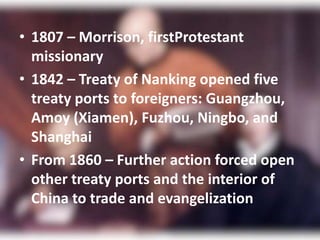The image is a poster depicting chronological events in China's history, adorned with white text bullet points at the center. In the blurred background, there's an old-style painting of three men, likely religious leaders or forefathers, two seated in dark suits and one standing in an orange gown, possibly traditional Asian attire. The poster's text features:
1. 1807 - Morrison, first Protestant missionary.
2. 1842 - Treaty of Nanking opened five treaty ports to foreigners: Guangzhou, Amoy (Xiamen), Fuzhou, Ningbo, and Shanghai.
3. 1860 - Further actions forced open other treaty ports and the interior of China to trade and evangelization.